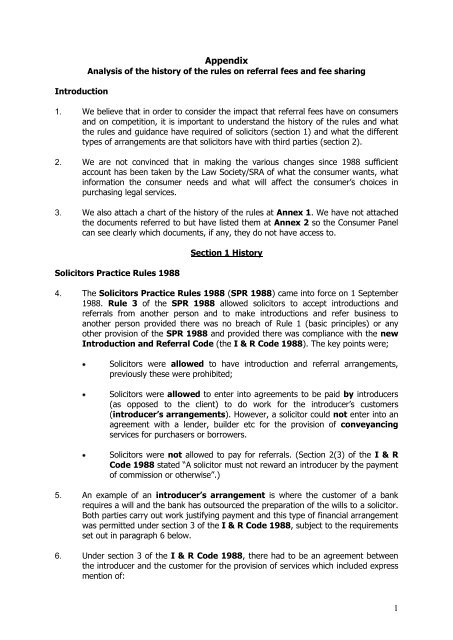This image captures a page from a book, with a white background and black text. At the top, the title "Appendix" appears prominently, followed by the bolded header "Analysis of the History of the Rules on Referral Fees and Fee Sharing." Beneath this, the introduction is presented with three numbered bullet points that delve into the impact of referral fees on customers and competition, questioning the adequacy of changes made since 1988 concerning consumer needs and preferences. 

The text transitions into "Section 1: History," which is underlined and introduces the "Solicitors' Practice Rules 1988." This section includes several detailed points: the rule allowed solicitors to accept introductions and referrals under specific conditions outlined in the rules and the Introduction and Referral (I&R) Code of 1988. It highlights that solicitors could receive payments from introducers instead of clients for certain services, except in cases involving lenders or builders. An example provided describes banks outsourcing will preparations to solicitors under permissible financial arrangements. 

The page number "1" is situated at the bottom right of the page.